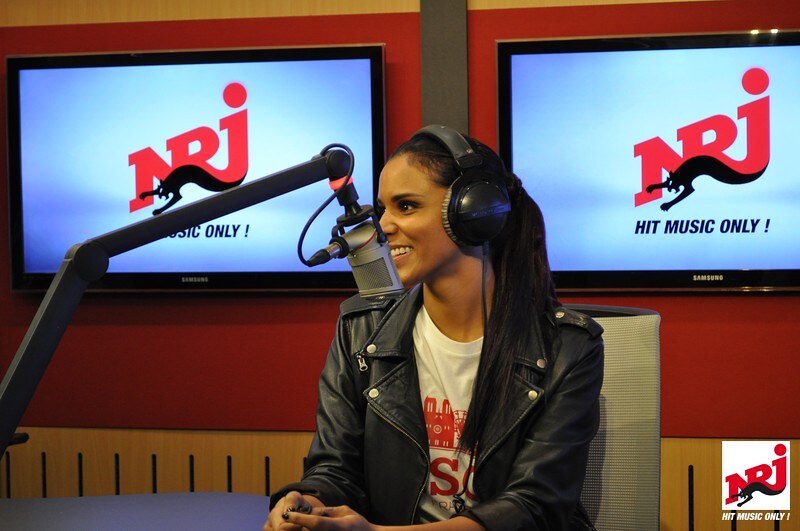In the image, we see a young black woman, potentially African American, seated at what resembles a radio show or broadcasting station. She is dressed in a white t-shirt featuring some red writing partially obscured by a black leather jacket adorned with buttons, which she wears with its collar popped open. She sports over-the-ear black headphones and her fingernails are painted black. Positioned directly in front of her is a whitish-silver microphone on a stand, extending from the bottom left corner towards her face. Her long, dark hair cascades down as she looks off cheerfully to her left, her broad smile revealing her teeth. In the background, against a red wall, there are two Samsung TV screens. Both TVs display the same logo: "NRJ" with a silhouette of a panther beneath it and the slogan "Hit Music Only." The same logo is visible in the bottom right corner of the image. The overall scene captures the dynamic atmosphere of a radio station with the woman evidently engaged in a lively broadcast.